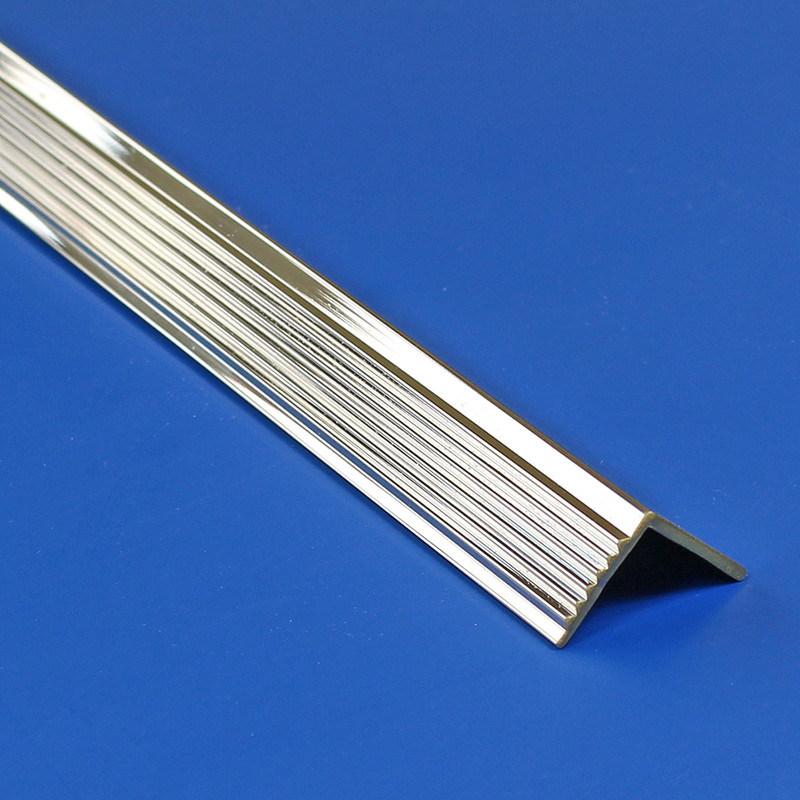The image depicts a shiny, silver aluminum L-shaped metal piece set against a blue background. The longer side of the L features six evenly spaced, raised ridges reminiscent of a running board on a car or the frets on a guitar. The shorter side is smooth. This piece, which could be described as an edging cover or trim, potentially serves various purposes such as protecting furniture corners, steps, or possibly even as a decorative element in automotive applications. Its sleek and polished appearance also suggests it might be used as a nameplate for desks or doors.